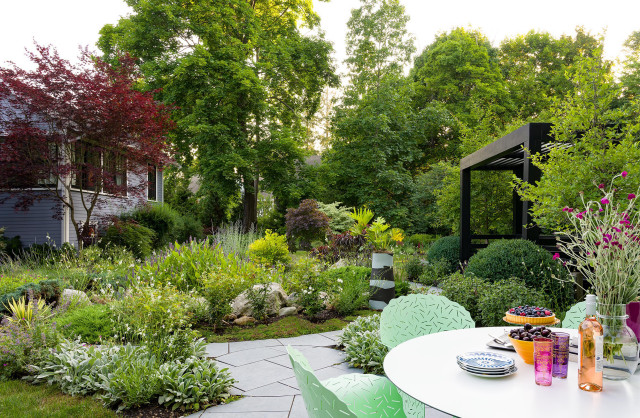The image showcases a meticulously maintained garden area adjacent to a blue-gray house with white pillars. In the foreground on the right, there's a concrete-paved patio with a circular white dining table. The table features stacked plates, a cheesecake adorned with berries, an orange bowl of round vegetables, two glass cups in magenta and purple, and an orange bottle. Surrounding the table are distinctive green, wrought-iron chairs with patterned openings. Bordering this scene are a variety of lush shrubs and flowering plants, which line a flagstone walkway leading to a wooden arbor. In the background, among the trees including a striking maple with reddish leaves, the house peeks through, completing this serene and inviting garden setting.